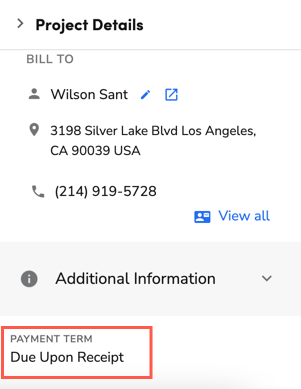The image is a screenshot taken from a mobile device, specifically showcasing project details. At the top of the screen, the text "Project Details" is prominently displayed in bold. Below this, the section labeled "Build To" contains an icon of a small person next to the name "Wilson Sant." Adjacent to the name, there is a pencil icon indicating the ability to edit this information, along with a pop-out icon for additional options.

Underneath this section, there is an address icon followed by the address: "3198 Silver Lake Blvd, Los Angeles, CA, 90039 USA." Directly below the address, a phone icon is present with the accompanying phone number: "214-919-5728."

To the right of these details, there is a blue link labeled "View All," presumably for accessing more comprehensive information. Further down the image, against a light gray background, an eye icon appears next to the text "Additional Information," which can be expanded for more details.

At the bottom of the screenshot, the payment terms are specified as "Due Upon Receipt," distinctly highlighted with a red rectangular box around this text.